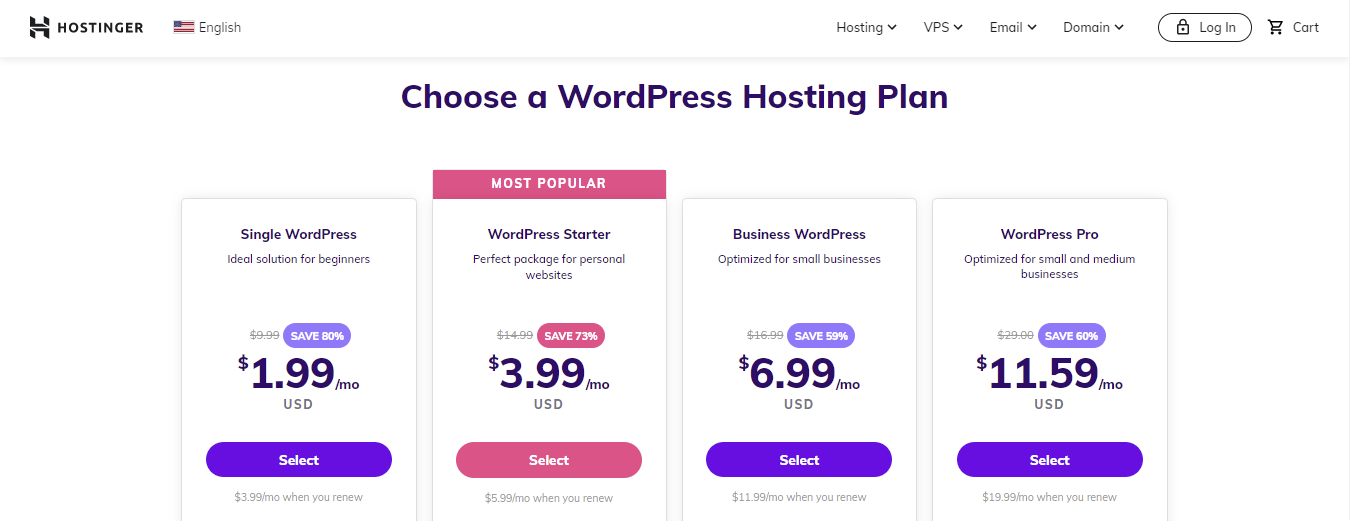This image is a screenshot of the "Choose a WordPress Hosting Plan" page on the Hostinger website. The background is predominantly white, providing a clean and minimalistic backdrop. 

At the top left corner, the Hostinger logo is prominently displayed, featuring a stylized 'H' followed by the word "Hostinger" in all capital letters. Adjacent to the logo on the right side is an icon of the US flag accompanied by the word "English."

To the right of this layout is a large space, proceeding to the website's navigation section, which is aligned to the right. The navigation menu features options in title case letters: "Hosting" (with a drop-down menu icon), "VPS" (with a drop-down menu icon), "Email" (with a drop-down menu icon), and "Domain" (with a drop-down menu icon). Following these options is a button with rounded edges labeled "Login," adorned with a padlock icon indicating security. This button has a black outline. The final icon is a shopping cart with the label "Cart" next to it.

Below this header area, a light gray border of approximately five pixels in width extends across the page, giving a slight drop shadow effect that adds depth. 

In the central part of the image, the heading "Choose a WordPress Hosting Plan" is displayed in bold, dark-colored letters, possibly black or dark blue, and written in title case.

Below the heading, there are four distinct plan tiles arranged from left to right:

1. **Single WordPress Plan**:  
   - Descriptive text explaining the details of the plan.
   - Price: $1.99/month USD, with information on potential savings.
   - A blue button at the bottom center, with rounded edges and the word "Select" in white letters.
   - Additional information in light gray text below the button.

2. **WordPress Starter Plan**:  
   - Topped with a maroonish-purple banner labeled "Most Popular" in white letters.
   - Descriptive text outlining the plan's features.
   - Price: $3.99/month USD, with details on savings.
   - A maroonish-purple button at the bottom center, labeled "Select" in white letters.

3. **Business WordPress Plan**:  
   - Oriented towards small businesses, as indicated by the subtitle.
   - A badge indicating "Save 60%".
   - Price: $6.99/month USD.
   - A maroonish-purple button at the bottom center, similar to the previous plan, labeled "Select" in white letters.

4. **WordPress Pro Plan**:  
   - Descriptive text underlining the advanced features of this plan.
   - Price: $11.59/month USD.
 
Each of these tiles provides users with a clear overview of the available plans, their prices, potential savings, and conveniently placed "Select" buttons for seamless navigation and selection.